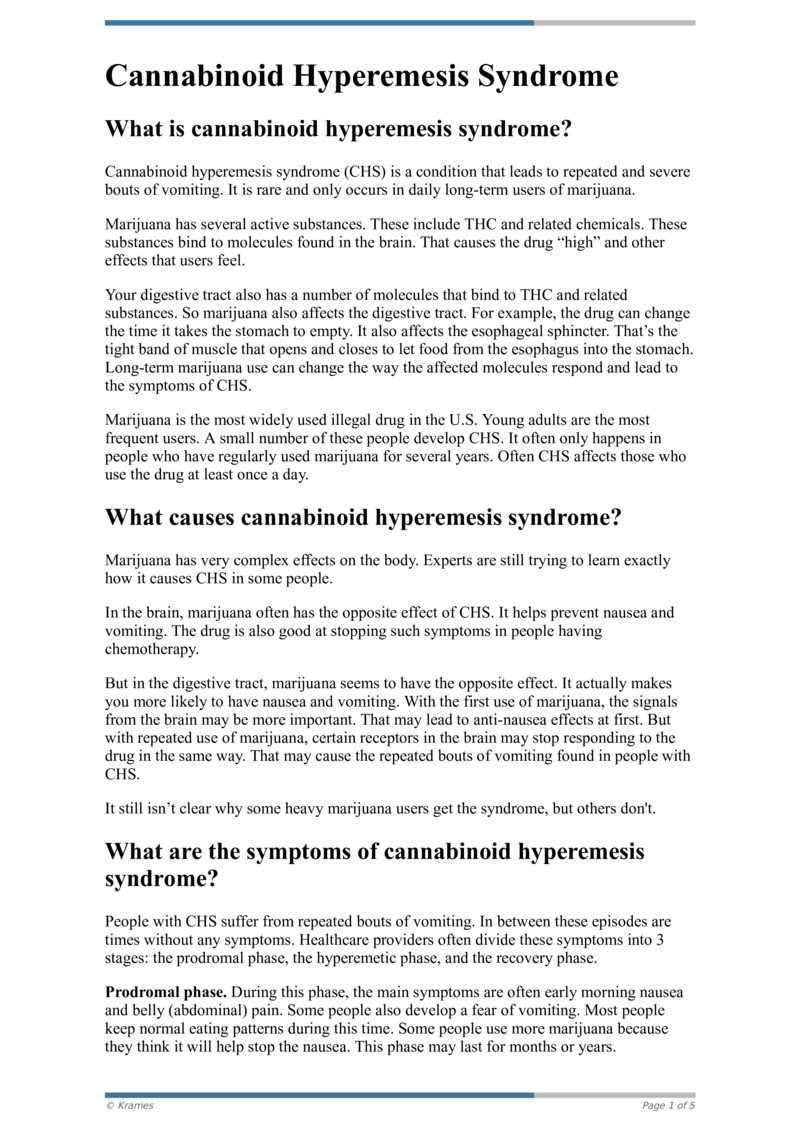This image features a comprehensive block of text that provides an in-depth definition and explanation of Cannabinoid Hyperemesis Syndrome (CHS). The text explains that CHS is a rare medical condition characterized by recurrent and severe episodes of vomiting. It primarily affects individuals who are daily, long-term users of marijuana. The text highlights that marijuana contains active substances, including THC and related chemicals, which interact with molecules in the brain and digestive tract. These substances bind to specific receptors in the brain, inducing the drug's high and other effects felt by users. Additionally, THC and similar compounds also interact with receptors in the digestive system, further influencing its functioning and contributing to the symptoms of CHS.